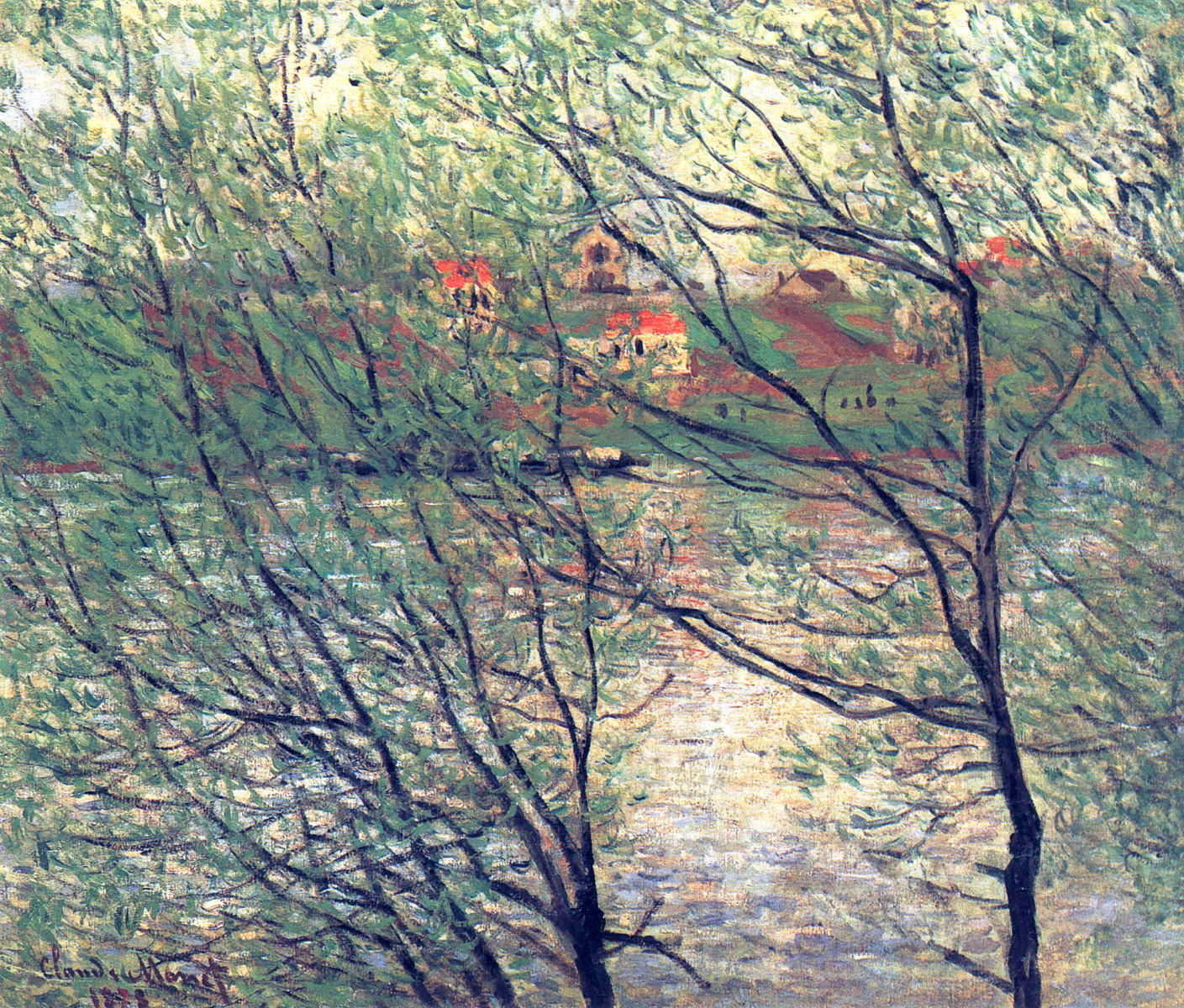An oil painting captures a serene outdoor scene from the perspective of someone positioned behind young trees, gazing out over a tranquil pond. The still water of the pond reflects an array of colors including blues, greens, and yellows, creating a mesmerizing mirror effect. Beyond the pond, the landscape gently rises to reveal a bank dotted with several houses. Prominently featured are three white houses with orange gabled roofs and a larger two-story brown house with its own gabled roof. Off in the distance, a windmill adds a rustic charm to the idyllic setting. The young trees in the foreground, budding with fresh leaves, suggest the onset of spring. The sky overhead is a light green, softly illuminating the gentle slope and the rich variety of colors in the scene. The painting, reminiscent of Claude Monet's impressionistic style, beautifully captures the harmony between nature and human habitation.